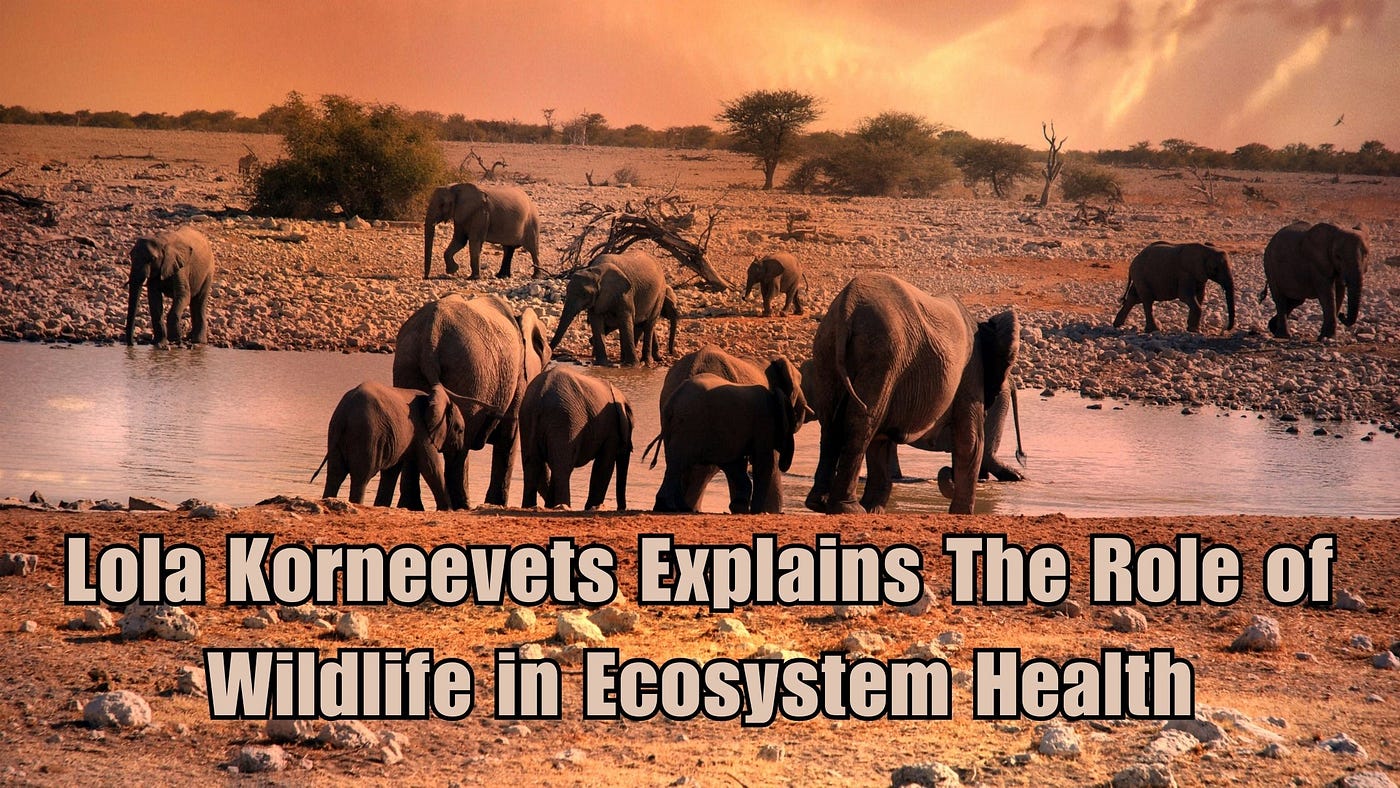In this captivating landscape photograph, a group of at least a dozen elephants roams the vast savannah, their figures standing out against a color filter that renders the scene in shades of orange, umber, and brown. Positioned around a sizable watering hole in the center, many of the elephants are drinking, their heads and trunks lowered in concentration. The ground, a mix of red soil, rocks, and gravel, stretches out beneath them, with dirt paths visible around the watering hole. In the background, sparse trees and green shrubbery dot the horizon under an orangish sky with few clouds. Bold white text at the bottom reads, "Lola Korniewicz explains the role of wildlife in ecosystem health," providing context to the tranquil yet purposeful activity of the elephants within their natural environment.